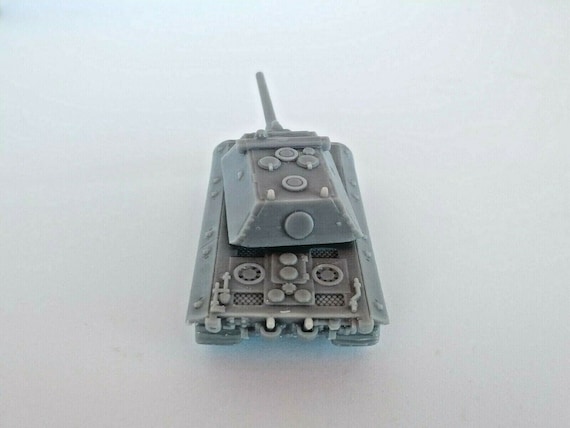This photograph features a small, unpainted gray plastic model of a military tank set against a plain white background. The tank has a trapezoidal shape with sharp, flat surfaces and a single gun barrel at the front, which is slightly aimed to the left. The top of the tank is detailed with several circular shapes or portals, some extending to the sides. Additionally, you can see the long, rotating treads at the bottom of the tank. The image appears to be taken from a high angle, showing both the top and the back end of the tank, giving the model a detailed, almost 3D-printed appearance.